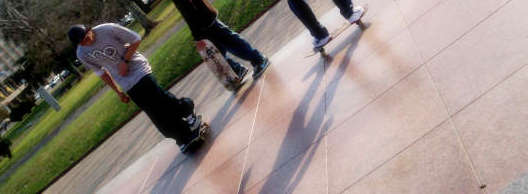The image captures an outdoor scene in what appears to be a park, featuring three skateboarders. The camera angle is tilted 45 degrees to the left. The setting includes large, light brown concrete tiles or squares, with manicured grass and a few trees in the background. A partially visible building sits in the far left corner, and sunlight is casting shadows from the upper right.

In the foreground, one skateboarder, wearing a hat and jeans, stands fully visible on his skateboard. To his side, only the lower half of another skateboarder is seen, with their skateboard propped against their leg; this board features a red and white design. On the right side of the image, a third skateboarder is seen from the knees down, with white shoes on their skateboard. All three appear relaxed in this open, public space.